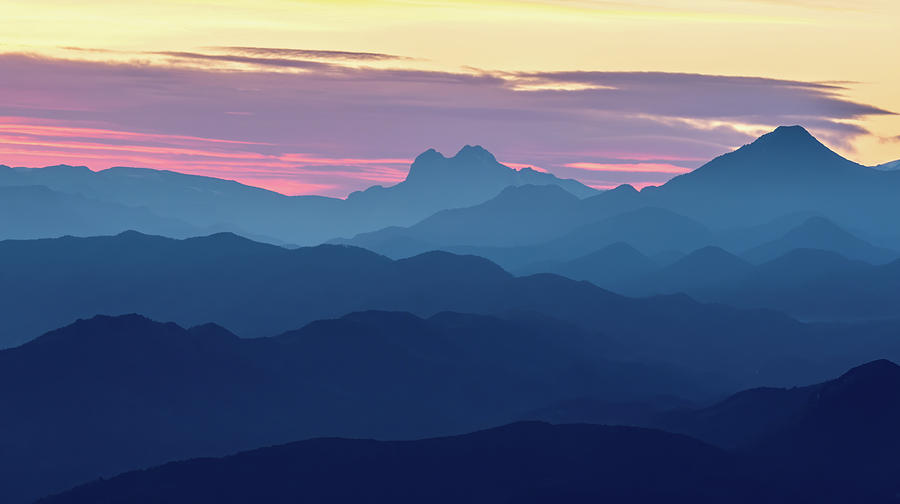In this detailed outdoor photograph, a series of mountain ridges unfold before us, each ranging in shades of blue that transition from deep, almost purple hues in the foreground to lighter blues as they recede into the distance. The mountains vary in height and shape, creating a layered effect with valleys interspersed between them. The furthest visible ridge showcases two peaks separated by a crevice, suggesting rugged and diverse terrain. Above these majestic mountains, the sky is alive with the colors of either a sunrise or sunset, displaying a gradient from bright pinks near the horizon to purples and light peaches higher up. Thick clouds are underlit with pink, orange, and darker purple tones, adding to the scene's dramatic beauty. The overall effect captures the serene yet striking isolation of the landscape, devoid of animals or people, and evokes a sense of cold tranquility amidst the grandeur of nature.